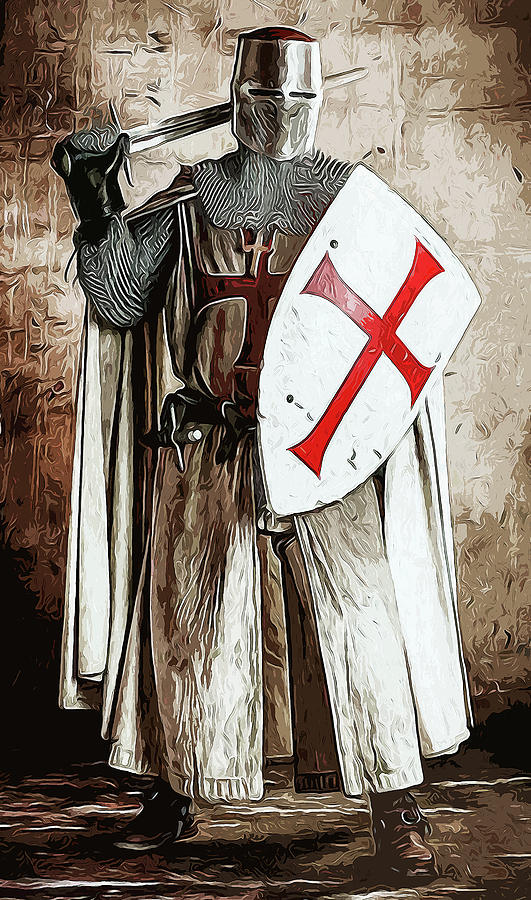This detailed painting depicts a medieval Crusader knight standing against a brownish, stone-like background that evokes the walls of a castle. The knight is dressed in chain mail and a cream-colored tunic featuring a prominent red cross across the chest, symbolizing his participation in the Crusades. His face is fully concealed by a square helmet with thin horizontal eye slits, lending an air of formidable anonymity. The knight's right arm is confidently raised, resting a sword over his shoulder, while his left hand grasps a large, tattered white shield adorned with a red cross. A dagger hangs at his waist, and around his neck, a cross pendant adds to his depiction as a warrior of faith. The scene is meticulously rendered, closely resembling a detailed linoleum print or a precise painting, with a dark, earthy floor contrasting the knight's imposing figure against the austere, tile-like wall in the background.